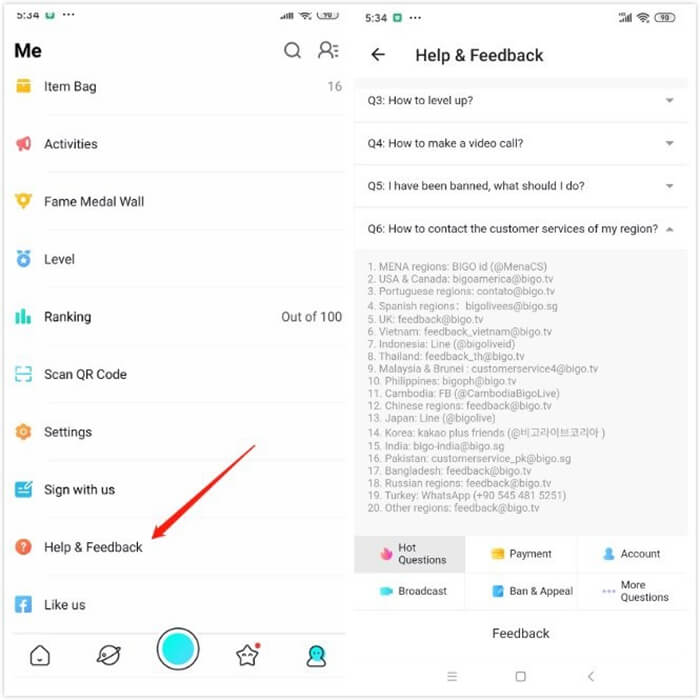The image displays a detailed user interface of an application, starting from the top left with a numeric indicator "534," followed by a row labeled "Me," beneath which are various navigation options including "Item Bag," "Activities," "Fame," "Metal Wall," "Level," "Ranking," "Scan QR Code," "Settings," "Sign with Us," "Help and Feedback," and "Like Us." Notably, there is a red arrow pointing specifically at the "Help and Feedback" option.

Below this section, there are several icons: a home icon, a circle with a check mark, another circle with a smaller blue circle inside, a star, and an additional unspecified icon.

To the right, the "Help and Feedback" section continues with several FAQs listed as Q3 ("How to level up"), Q4 ("How to make a video call"), Q5 ("I have been banned, what should I do"), and Q6 ("How to contact the customer services of my region"). 

Further down, grouped under the "Hot Questions" category, there are links for "Broadcast," "Payment," "Ban and Appeal," "Account," and "More Questions." Centered at the very bottom of the interface is the "Feedback" option.